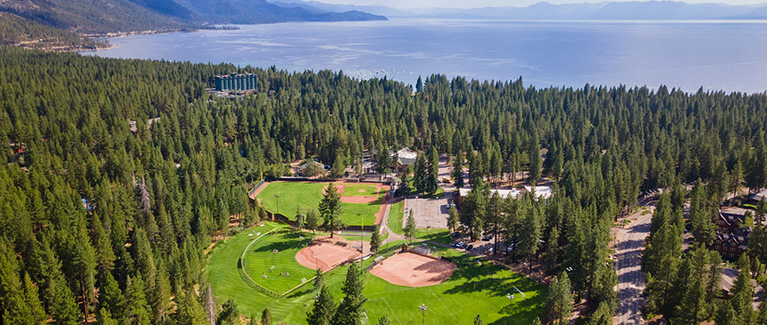This is an aerial view of a coastal area and its surroundings. The bottom three-quarters of the image showcases a lush, green region dominated by trees, ball fields, and a few structures. Starting from the top, a large body of slate-blue water extends across the image, flanked by distant landmasses, possibly mountains, in the far distance. The top left of the image reveals a stretch of land hugging the coast, transitioning into a dense tree line separating the water from the inland area. 

On the left side, amidst the thick foliage just below the prominent tree line, there appears to be a notable building, potentially a restaurant, enveloped by trees on all sides. Extending horizontally, the tree line gives way to a verdant area dotted with three neatly aligned baseball or softball fields. These fields span from just left of center towards the bottom of the image, each showcasing fences and parking areas indicative of a designated recreational zone for multiple teams to play simultaneously.

A road meanders upward from the bottom right corner, flanked by trees, before curving off to the right, adding a sense of seclusion to this private, greenery-engulfed recreational area. The scene is framed by additional clusters of trees at both the bottom and right edges, enhancing the picturesque blend of natural beauty, water, and organized play areas.